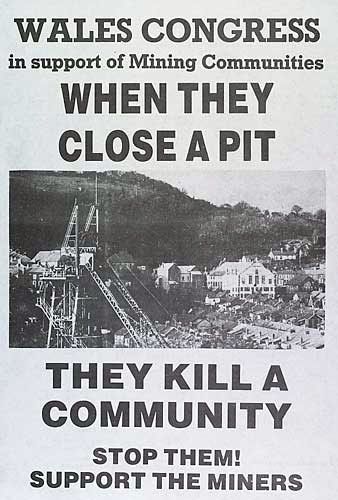This black-and-white promotional flyer is an advocacy piece from the Wales Congress in support of mining communities. Dominated by text in all capital letters, it urgently proclaims: "WHEN THEY CLOSE A PIT, THEY KILL A COMMUNITY. STOP THEM! SUPPORT THE MINERS." The central section of the flyer features a blurred black-and-white photograph depicting a mining town. The image shows a contemporary mine with various structures and buildings, including some houses with gabled roofs and a hill in the background. Ladders can be seen ascending one of the mine structures, while trees frame the scene, emphasizing the industrial and residential aspects entwined in the life of the mining community.